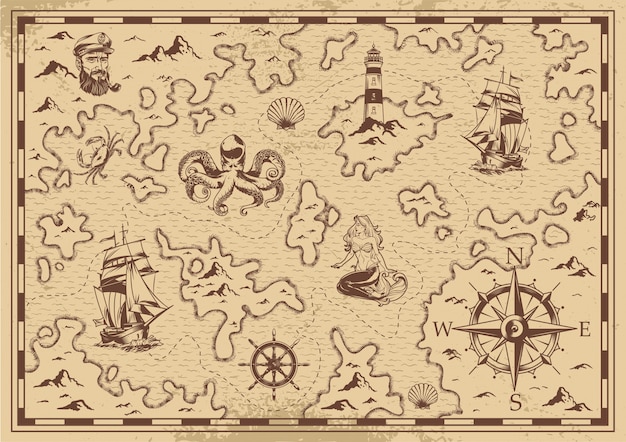The image depicts a square, light tan treasure map with a darker brown border and various detailed drawings scattered across it. In the upper left corner, there is a man's face with a captain's hat, complete with a beard and mustache, set against a backdrop of mountains. Below the captain, a crab can be seen, followed by a sailboat further down. The map features numerous islands and landmasses drawn throughout. Key elements include an octopus, a seashell, and a steering wheel of a ship near the bottom left. Prominently in the center stands a lighthouse and a mermaid. In the bottom right corner, there's a compass marked with north, south, east, and west. The top right corner showcases another sailboat, with visible dashed lines connecting various points around the map, providing a sense of direction and journey.